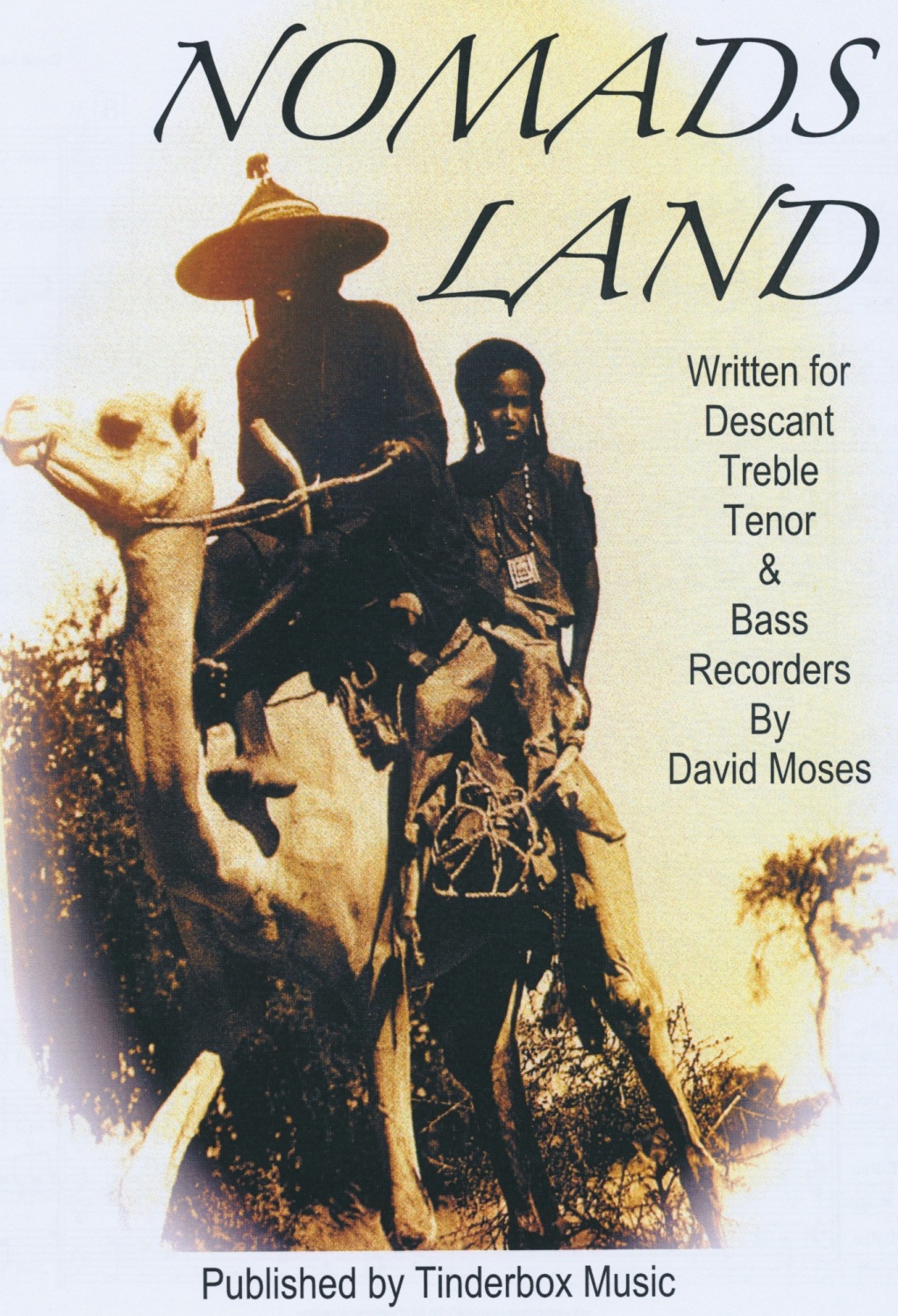The image, taken outdoors during the daytime, serves as the cover of a music piece titled "Nomad's Land." It features two people in traditional garb riding on the same camel. The person in the front, whose face is completely obscured by a wide-brimmed hat, appears to be in the shade. Behind them is a younger female with dark hair. The title "Nomad's Land" is prominently displayed at the top, with additional text on the right side that reads, "written for descant, treble, tenor, and bass recorders by David Moses," and at the bottom, "published by Tinderbox Music."